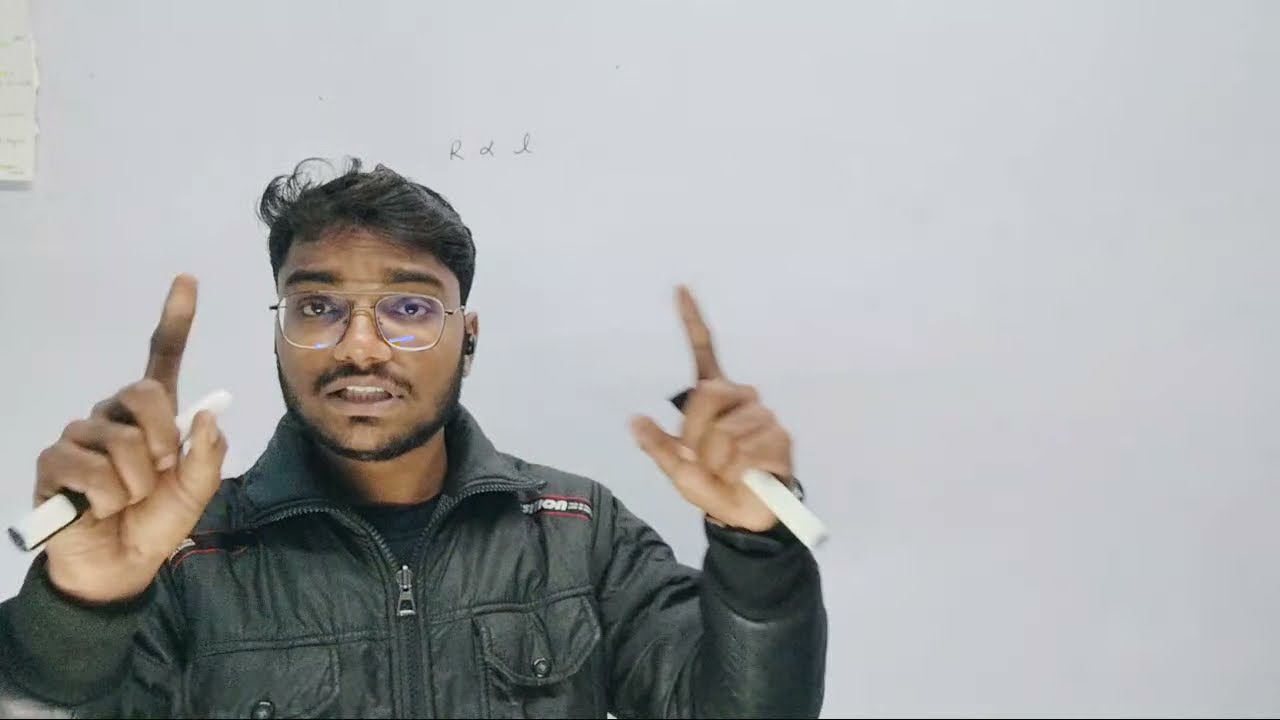In this photograph, a man, positioned primarily on the left side of the image, appears to be teaching or explaining something. He is in motion, with both hands raised in front of him, gripping what look like white markers. His index fingers and thumbs are prominently pointed upwards. The man's features include dark hair styled to swoop at the front, bushy brown eyebrows, a beard, and a mustache. He also sports square-framed glasses, and an earbud can be seen in one of his ears. He is dressed in a black bomber jacket with two front pockets on each side, worn over a black t-shirt.

In the background, a whiteboard displays the capital letters "R" and "L," with the "L" written in cursive. To the upper left, layered pieces of paper are visible. The main focus of the image is on the man's face and his right hand, with his left hand appearing slightly blurred. The overall scene suggests he is engaged in a teaching or explanatory gesture against a backdrop of an otherwise minimalistic setting.